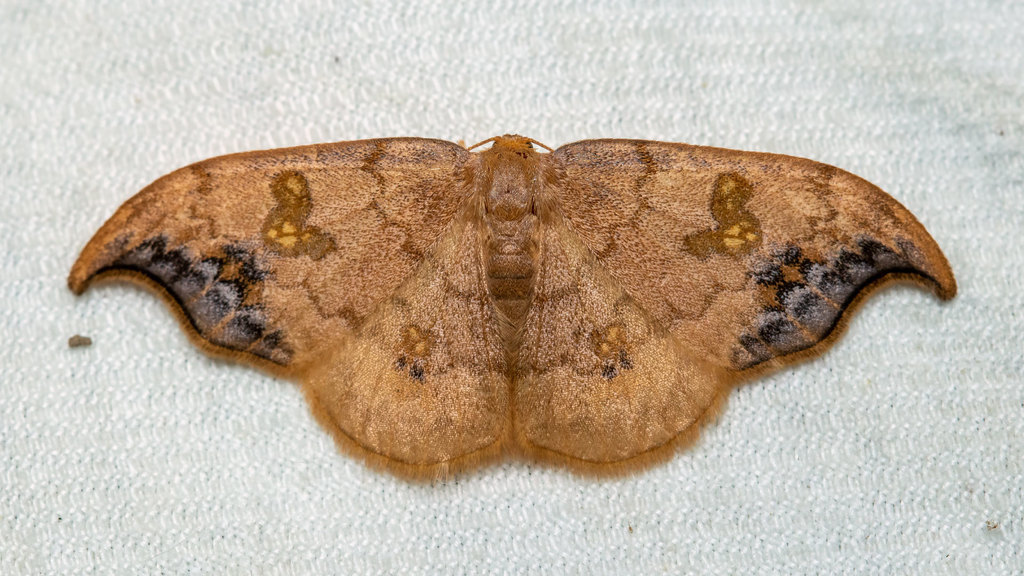The image depicts a brown butterfly, possibly deceased, meticulously laid out on a light gray, patterned fabric surface, resembling a white cloth. The creature is positioned symmetrically, with its wings fully expanded and its back facing the camera. The wings are adorned with dark brown and light yellow splotches, creating a striking contrast. Along the edges of its wings, darker patches, or plaque, add to the intricate design. The edges of the wings feature a curved, wavy pattern. This photograph appears to have been taken indoors, suggesting the setting could be a doctor's office, a veterinarian's office, or perhaps a book collector's environment.